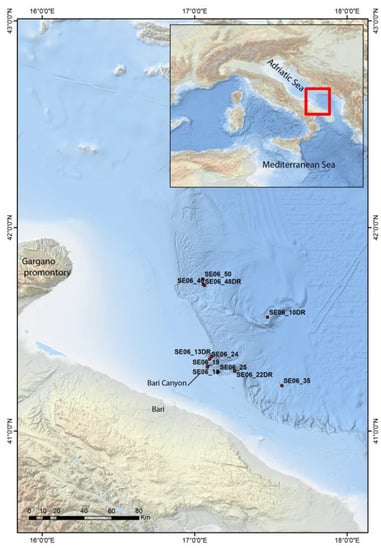This is a vertically aligned rectangular image resembling a map with a black border around its edges. At the top right corner, there is a smaller, bordered inset map showing a portion of Italy and Greece, with annotations reading "Adriatic Sea" and "Mediterranean Sea." A small red square is drawn slightly to the right on the map, indicating a specific highlighted area. Around the edges of the main map, there are several location coordinates in black text.

The upper portion of the main map is predominantly blue, representing the sea, while the lower part features various shades of brown and tan, depicting land. This differentiation between land and sea is clear, with the Adriatic Sea situated centrally and a brown landmass labeled "Gargano Promontory" towards the left middle section. Additionally, blue and white hues near the top and light green to brownish color lower down further denote the varying terrains from sea to shoreline.

The map contains numerous small black text descriptions, numbers, and dots, including "SE0413DR" and the words "Berry Canyon" in the blue water area. At the very bottom left corner, there is a legend with a black strip and numerical markers to indicate distances, marked with the "KM" symbol. The intricate detailing of coordinates and placement of the Adriatic and Mediterranean Seas provides a comprehensive depiction of this geographic area.